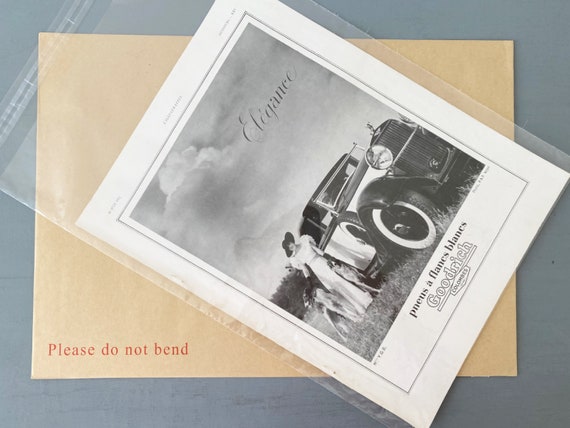The image features a black and white photograph set against a medium gray surface. The photograph is encased in a cellophane bag and depicts an old-style car, predominantly black with white accents. Standing next to the passenger side of the car is a woman dressed in a long white dress and a black hat, holding two dogs that reach about hip height. Above the scene, the word "Elegance" is printed, seemingly in the clouds. At the bottom of the photograph, the caption reads "Goodrich Colonists" and further below, "PNEUS A FLAMES BLANCS." The photograph is accompanied by a tan envelope lying behind it, labeled "Please Do Not Bend."